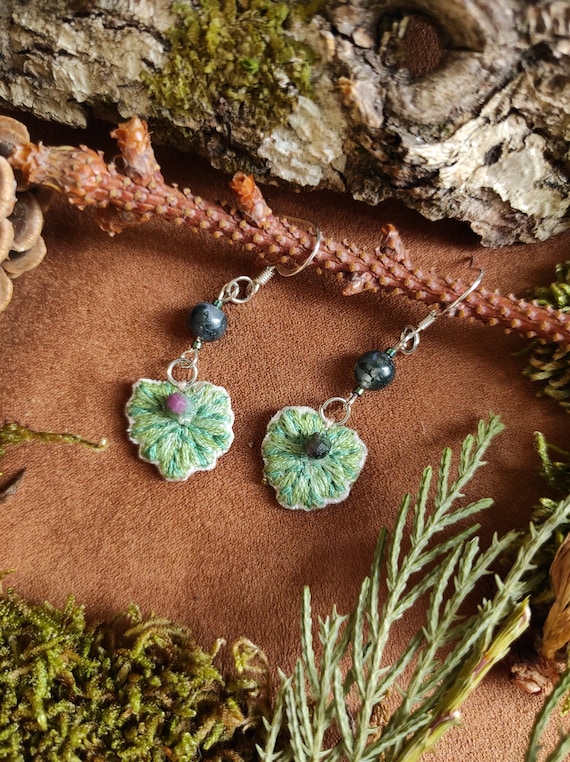This photograph features a pair of handcrafted, leaf-shaped earrings displayed in a naturalistic setting that might be intended for an Etsy listing or similar. The earrings are suspended from a gnarled pine branch, which stretches horizontally across the center of the image. The hooks, possibly made of silver, are connected to the main body of the earrings by wrapped wires and a series of beads. The beads include a black or dark blue one, and another that appears to be clear plastic or glass. The earrings themselves are crafted from different shades of green crochet, each adorned with a small gem—pink in the center of the left earring and green in the center of the right earring, giving the appearance of a leaf with a central button or ball. The background features a sandy ground, with a rock at the top adorned with patches of moss. Additional natural elements include a pine cone off to the left and various pine needles. In the top right corner, a plant extends out of the frame, enhancing the natural ambiance of the scene.